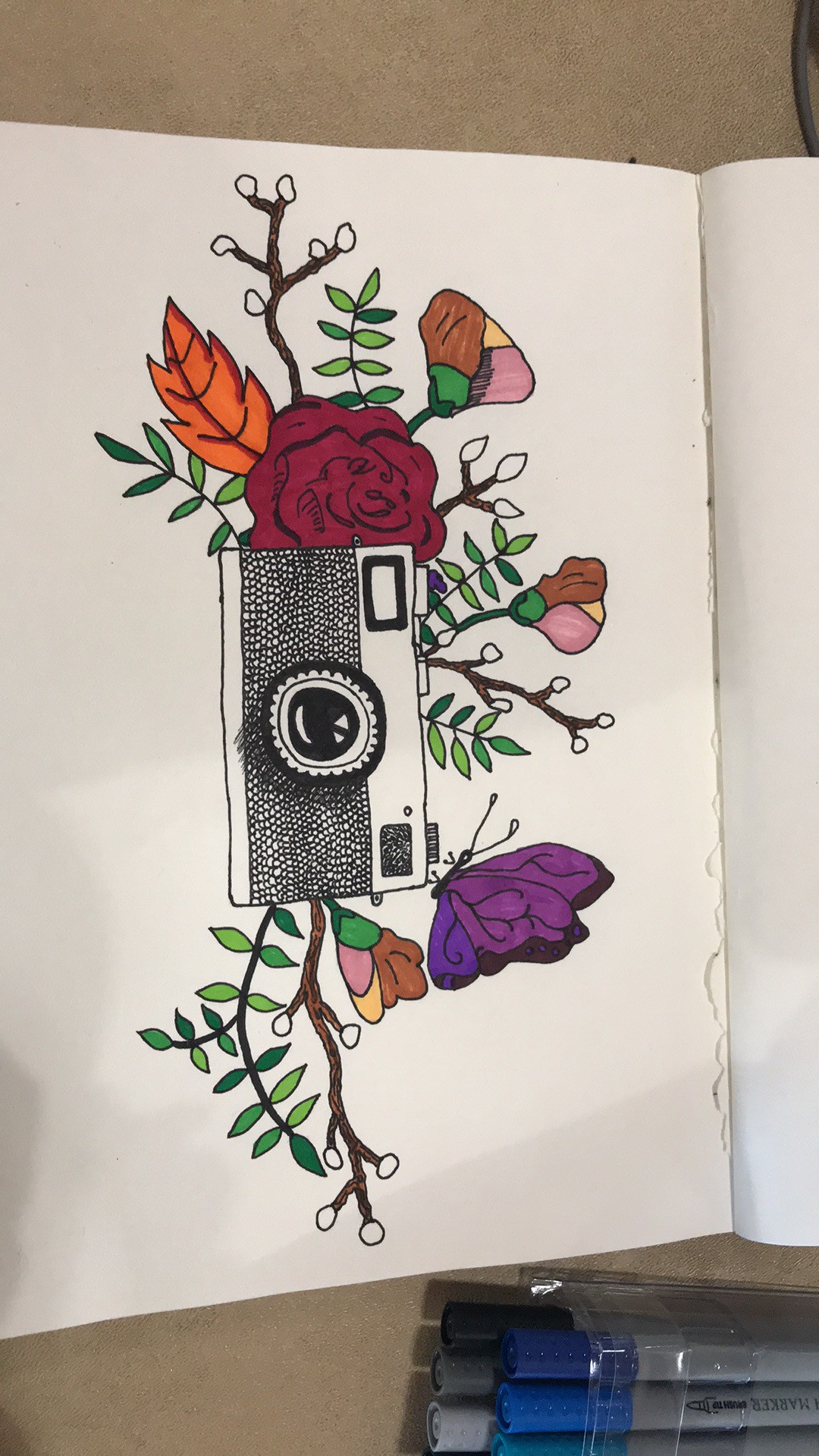The image showcases an open sketchbook lying on a brown table, revealing an intricately drawn and colored picture of an old-fashioned camera. The camera, sketched in black ink and detailed with markers, evokes a sense of vintage charm with its circular lens and buttons. Surrounding the camera are vibrant floral elements, including a large red rose, delicate baby breath, and various branches adorned with leaves of different shades—dark green, light green, and multicolored ones resembling ice cream hues of green, pink, yellow, and brown. Enhancing the scene's liveliness, a dark-to-light purple butterfly is seen perched on the upper left corner of the camera. On the lower right corner of the table, a plastic bag contains markers in various shades of purple and gray, indicating the tools used by the artist. This creative composition not only illustrates the camera but also breathes life into it with botanical and floral motifs, reflecting the artist's passion for photography and rendering it as a beautiful piece of art.